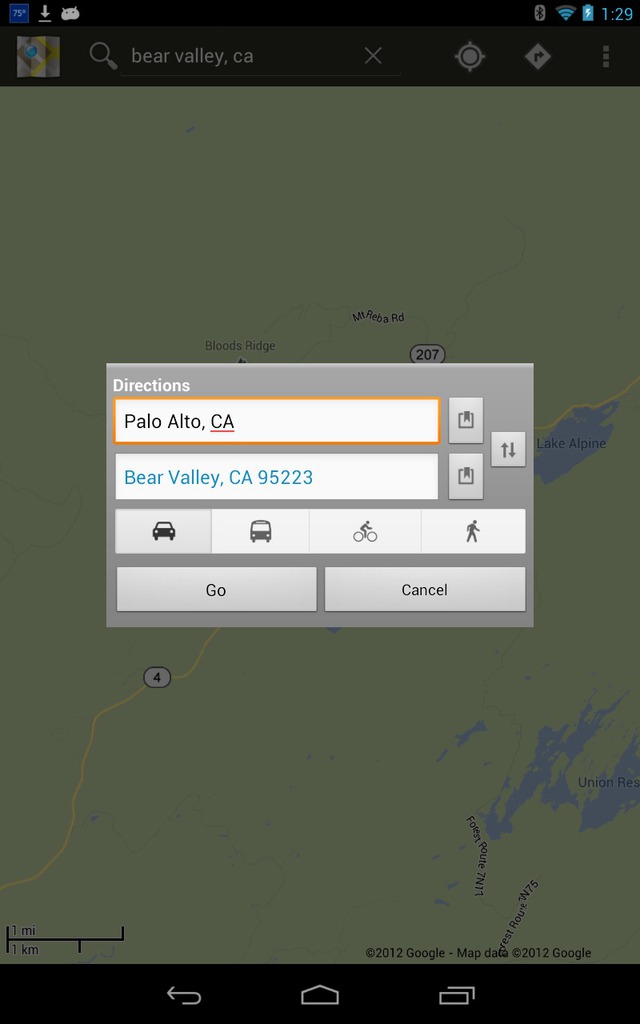The image depicts a smartphone displaying a map application. At the top, beneath the search bar, the location "Bear Valley, California" is indicated, complete with directional markers such as north, south, and a compass icon, along with an arrow pointing to the current orientation. In the background, a map is visible, showing a high-level view of the area.

Prominently in the foreground, there are input fields for generating directions. The starting point is "Bear Valley, California 95223," and the destination is "Palo Alto, California." Below these fields, there are travel mode options including car, bus, bike, and walking, along with buttons labeled "Go" and "Cancel."

Currently, the directions to Palo Alto, California have not been started, as the "Go" button has not been pressed, so the estimated travel time and step-by-step directions are not yet displayed. At the bottom of the screen, options are available to either save the current directions or start a new search by clicking a back button.

Though the interface and layout suggest it is a map application designed for mobile use, it does not resemble Google Maps. A tiny clock in the upper left corner reads 1:29, and there is also an icon indicating the option to download information.